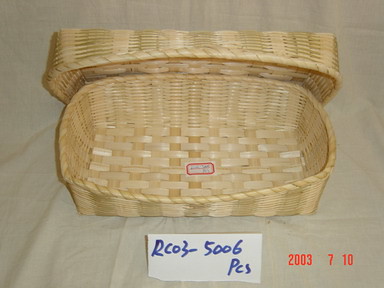The image is a small square photograph set against a pale, primarily white background, likely a sheet or cloth, featuring visible wrinkles and creases. Dominating the center is a light brown, tan, and black wicker basket, crafted from thin rods of wood in an under-and-over weave pattern. The basket has arched walls, and its wicker lid is seen leaning against it, positioned diagonally and upside-down. On the base of the basket, a red-bordered sticker is adhered, though its content is not specified. Additionally, there's a white slip of paper with blue text placed beneath the basket, which reads "RCO3-5006 PCS." Overlaying the photograph, in red lettering, is the date "2003 7 10," spaced unevenly across the bottom right of the image.